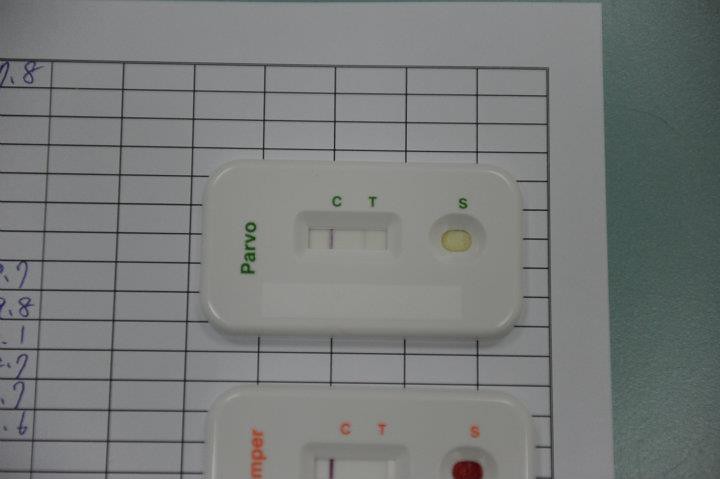The image depicts two medical test kits placed on a white paper that features a black grid. The grid is divided into eight visible columns and approximately 14 rows. The column on the far left contains some partial, yet discernible, numbers. The top test kit is fully visible, presenting as a white rectangle with rounded corners. Along the left side of this kit is the word "PARBO," printed vertically from bottom to top. The center features a view window with two horizontal lines, labeled "C" and "T." The line marked "C" appears darker than the one marked "T." To the right of the view window is a round indentation labeled with an "S," containing a drop of golden fluid. The bottom test kit displays a different brand name in orange text, although the name is partially cut off. Similar to the top test, the "C" line is darker than the "T" line. The "S" indentation on this kit contains a drop of red fluid.